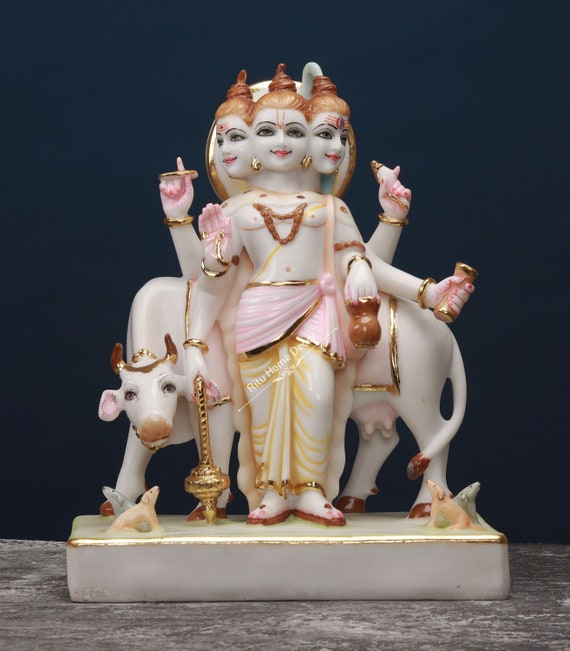This detailed image depicts a porcelain figurine on a rectangular base, which has a predominantly white color with gray streaks, a pale yellow front, and gold accents along the edge. The scene features a three-headed, six-armed woman standing in front of a white cow with brown-tipped features and horns, which is adorned with a gold crown. The woman has brown spiral hair styled like soft-serve ice cream, light-colored skin, and wears a layered outfit with a pink outer wrap and a white dress beneath it. She holds a gold object resembling an anvil. Small dogs are positioned at the cow's feet. The backdrop is a solid dark navy, while the base rests on a gray, weathered tabletop. The bottom-most part appears to have a wood-like, grayish color.